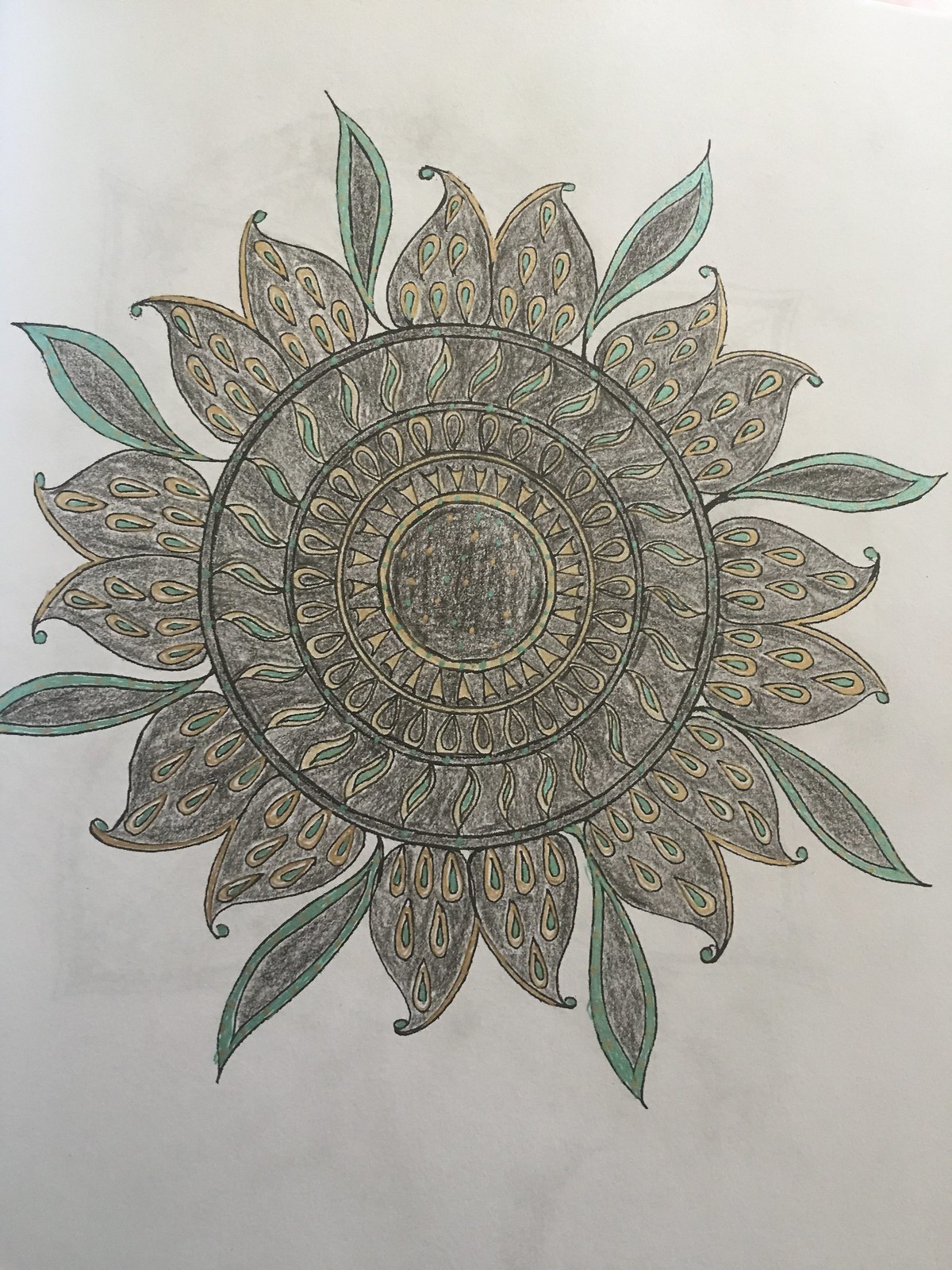This image features a detailed drawing that appears to be a cross between a mandala and a flower, created primarily with pencil and colored pencils. Set against a white, slightly beige background, the artwork is composed of concentric circular patterns starting from a central, fully shaded circle done in pencil. Surrounding this center are multiple rings, each adorned with intricate leaf-like designs. The first ring after the center includes touches of yellow beneath the leaves, followed by another ring with similar yellow highlights. The subsequent ring returns to being entirely pencil-shaded. Further out, the outermost ring displays elaborate flower petals, each containing tiny yellow raindrop-shaped details and occasional hints of green. The artwork is characterized by a palette dominated by gray and beige tones, with intermittent spots of yellow and green, bringing subtle yet striking accents to the piece. The meticulously colored work, resembling something from a high-end coloring book, presents a harmonious blend of precision and creativity with no text or other elements distracting from its intricate beauty.